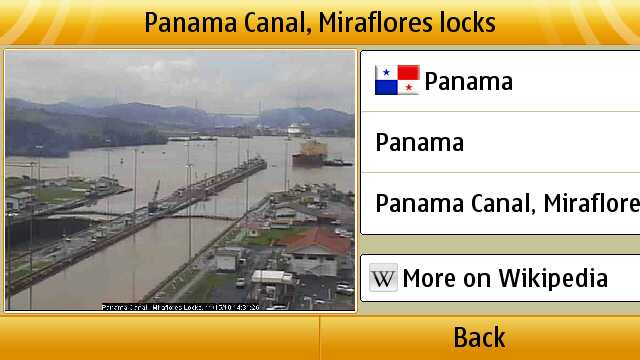This is a detailed screenshot of a webpage showcasing the Panama Canal's Miraflores locks:

**Upper Section:**
- At the top, there is a golden bar which contains black text reading "Panama Canal Miraflores Locks."
- Below this bar is an image framed within the page, displaying a panoramic view of the Panama Canal with mountains in the background and the canal water flowing between several structures on both sides.

**Middle Section:**
- Alongside the image, towards the right, is a series of hyperlinks. 
  - The first link is labeled "Panama" and is accompanied by the Panamanian flag. The flag is divided into four quadrants: the top-left and bottom-right quadrants are solid white with a blue star in the top-left quadrant and a red star in the bottom-right quadrant; the top-right is solid red, and the bottom-left is solid blue. 

**Lower Section:**
- Another golden bar at the bottom features the text, "Back" in the center.

**Additional Links:**
- Beneath the "Panama" link are additional links labeled "Panama Canal" and "More on Wikipedia," the latter featuring the iconic 'W' logo of Wikipedia.